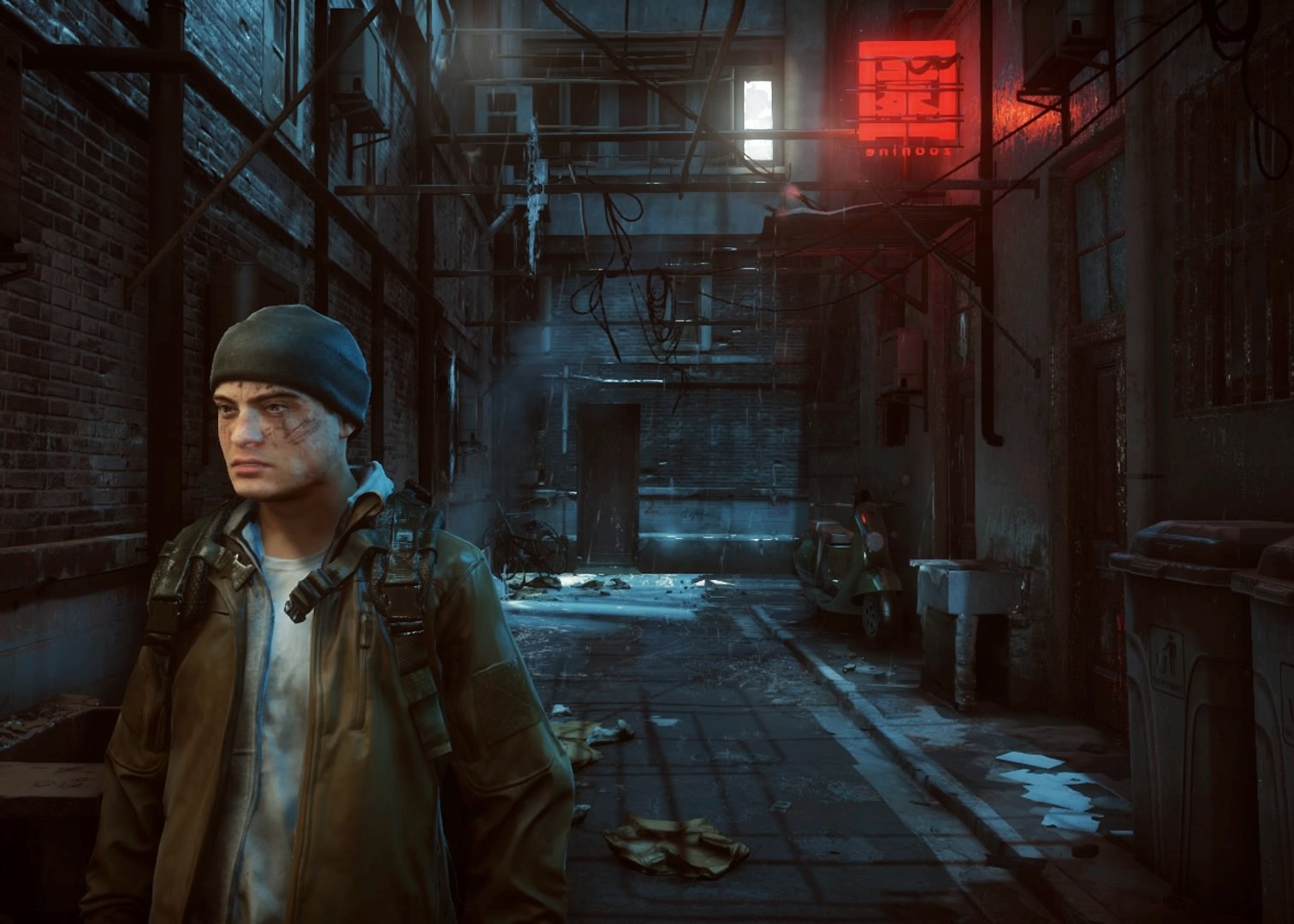In this color image, presented in the style of a computer game screenshot, we find ourselves in a dimly lit, indoor setting that likely resembles the interior of a warehouse. On the left side of the frame, a male figure is visible from the waist up, looking towards the left. He dons a black, snug-fitting stocking cap, and his face shows signs of grime, with dirt visibly smeared beneath his eye. On his nose appears to be a conspicuous white powder. The man is clad in a rugged brown jacket featuring various straps and fastenings, hinting at a utilitarian design. Beneath the jacket, he wears a white shirt marred by noticeable dirt smudges, completing his rough, weathered appearance.